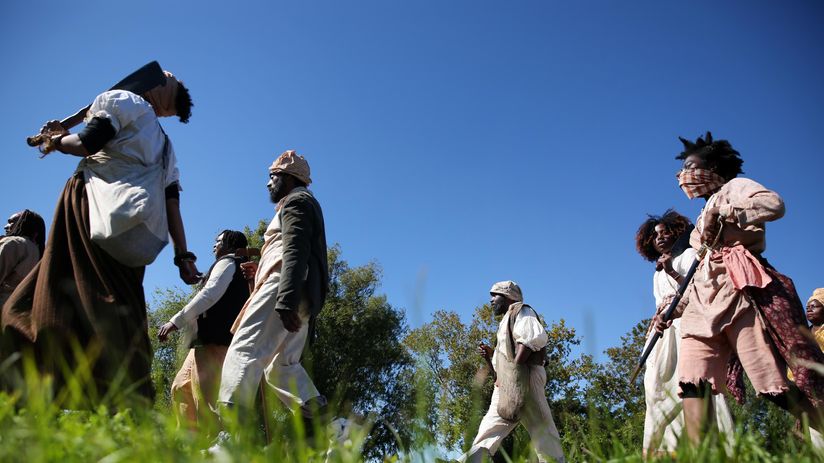In this striking outdoor photograph, the viewer is given a low-angle perspective, as if lying in the grass and looking up at a group of dark-skinned individuals walking through the scene. The bottom of the image is framed by out-of-focus blades of grass, while a vibrant, cloudless blue sky spans the top. A backdrop of distant trees adds depth to the setting. The group comprises both men and women, some with distinct hairstyles like dreads or braids, and a few carrying visible items such as a sword, club, or bags. 

Prominent within the image, a woman at the forefront, donning pink shorts and a pink top, conceals her nose and mouth with a bandana. Nearby, another woman in white with voluminous hair stands, partially obscuring a rotund woman in the background. The men, distinguishable by their hats, one in a dark shirt and white pants and another in a white shirt and white pants, are also present in the array of figures. They appear to be unified in their direction, walking towards the left, a collective yet individual tapestry of personalities and attire set against a natural, serene environment.